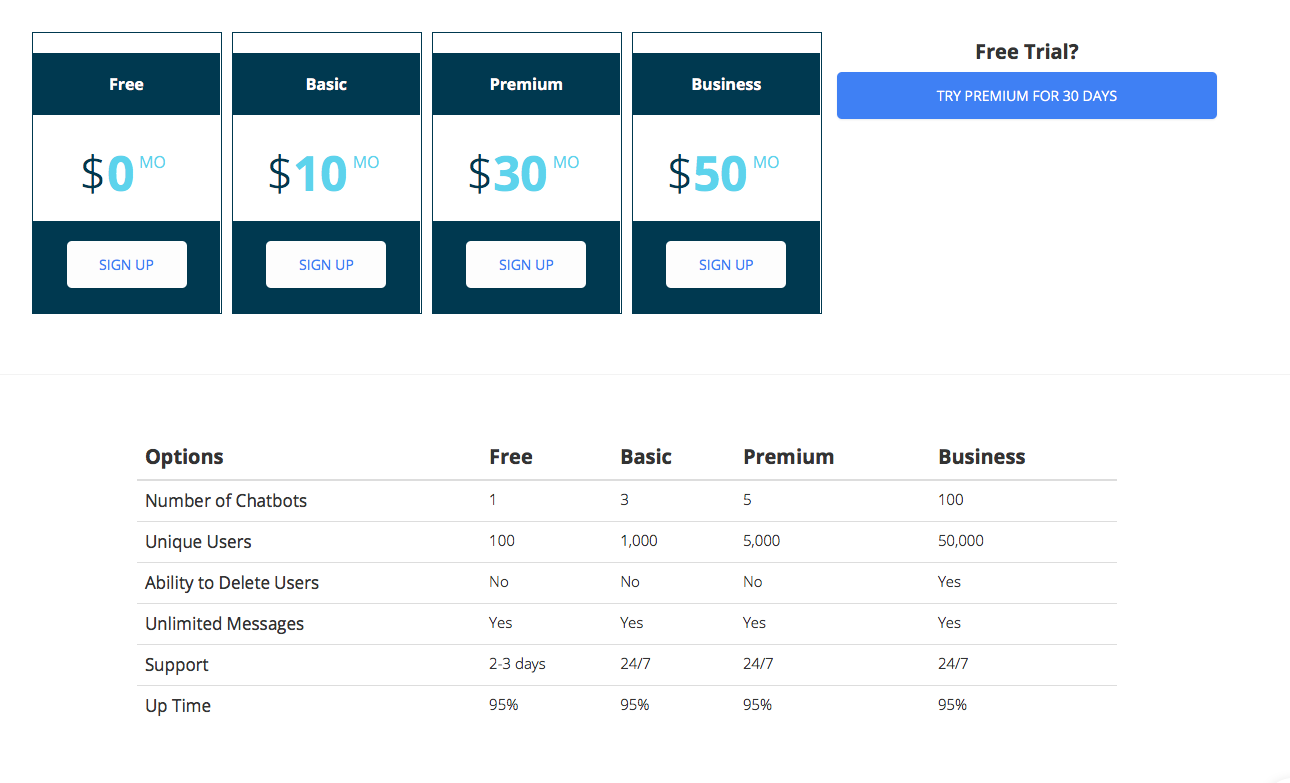The image depicts a webpage showcasing a tiered pricing structure for a service, offering multiple subscription options. The page has a clean, white background and features four vertical, rectangular boxes, each representing a different plan. Each box has consistent design elements: a dark blue header with white text indicating the plan name and pricing, and a navy blue footer with a white bubble containing light blue text that reads "Sign Up."

The four subscription options are as follows:
1. **Free**: Priced at $0 per month.
2. **Basic**: Priced at $10 per month.
3. **Premium**: Priced at $30 per month.
4. **Business**: Priced at $50 per month.

To the right of these options, there is an incentive for new users: "Free Trial: Try Premium for 30 days."

At the bottom of the page is a detailed comparison table with five columns and six rows. The columns list each plan—Free, Basic, Premium, and Business—while the rows specify the services or features included in each plan. These features include:
- Number of chatbots
- Unique users
- Ability to delete users
- Unlimited messages
- Support
- Uptime

Specific details about what each plan includes are provided under each column, allowing users to easily compare and determine which plan best suits their needs.